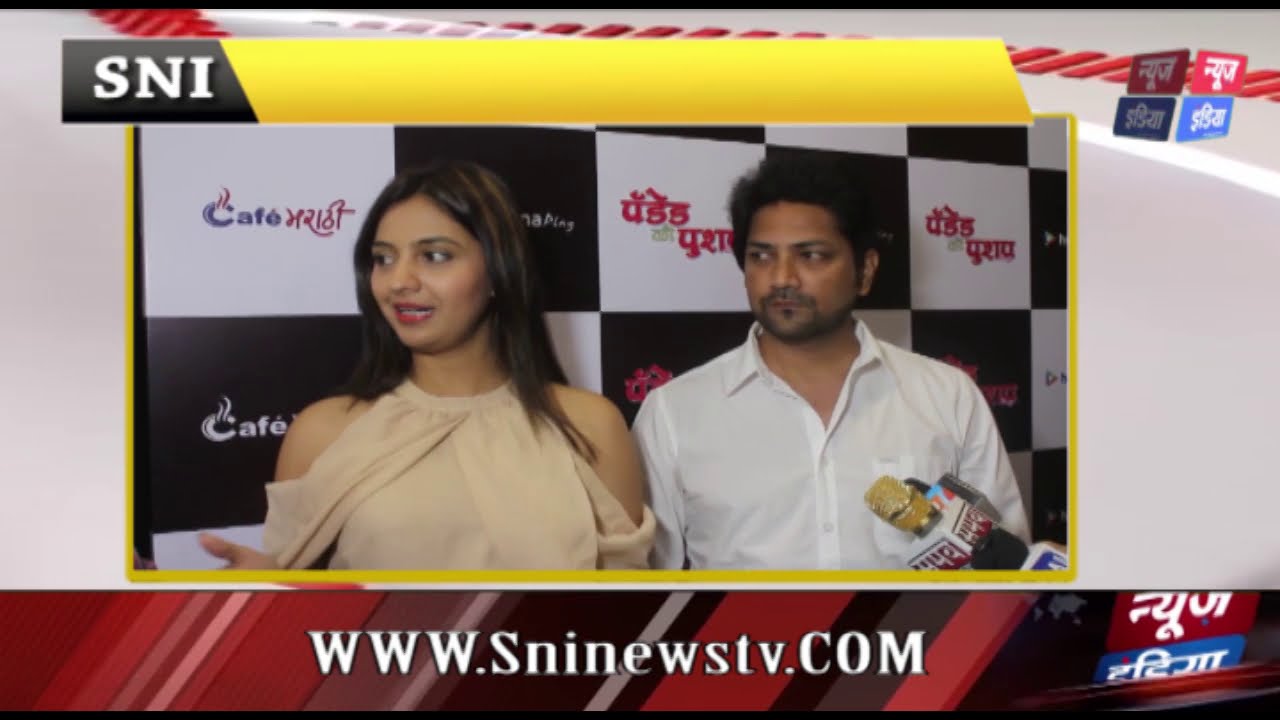This horizontal rectangular image appears to be a screenshot from a news broadcast. It features a man and a woman standing in front of a black and white checkered wall adorned with various sponsor logos, including "Cafe Riots" and "USS" (with the rest of the name unclear). The man, positioned on the right, has short black hair and a thin mustache and beard, and is dressed in a long-sleeve white button-down shirt. He has a serious expression and is looking off-camera to the right, where a microphone with a gold tip and a media station label is directed towards him. The woman, on the left, has long straight brown hair with highlights. She is wearing a sleeveless beige top that shows her shoulders and has a high neckline. She appears to be mid-speech, with one hand raised, and is also looking to her right. Both individuals are brown-skinned and appear to be captured in a candid moment during their broadcast.

The top of the image shows the caption "SNI" in white on a black backdrop, accompanied by a yellow chevron and a logo, suggesting the name of the news station or network. The bottom of the image features a border with the website "www.sninewstv.com" written in red, positioned against a background of diagonal red, black, and gray lines, further emphasizing the newsy nature of the production.